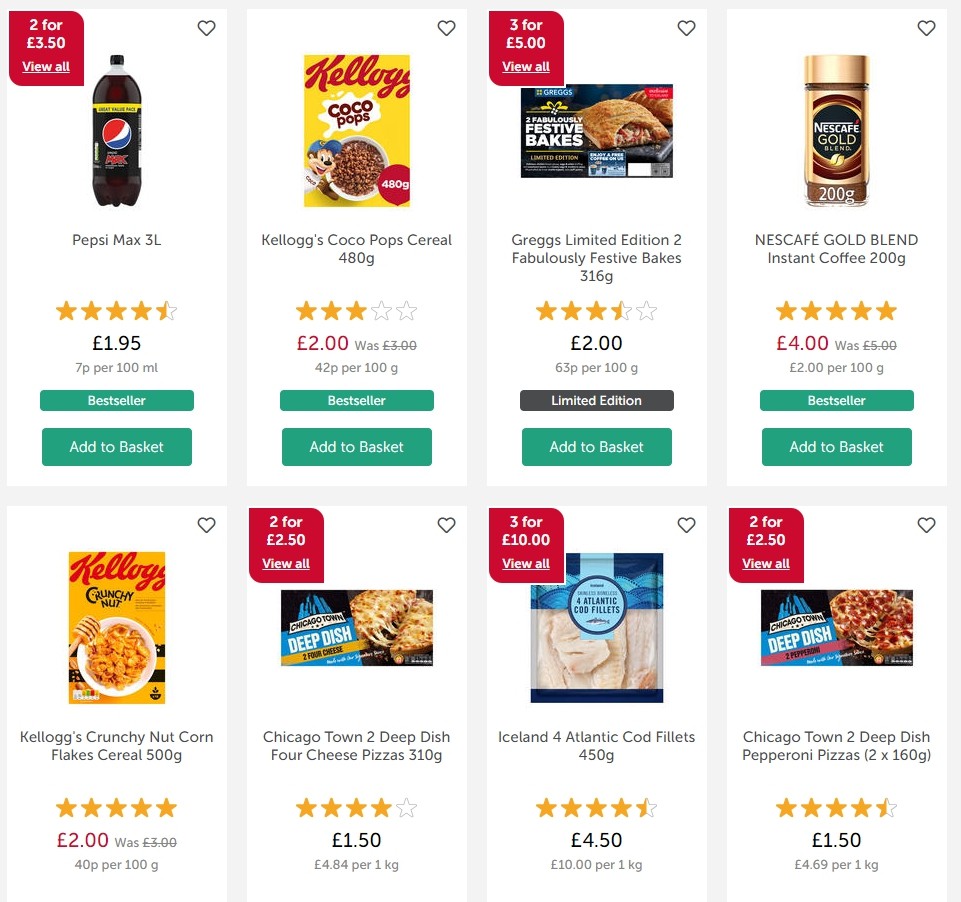The image displays a selection of food products, accompanied by British pound pricing. The products include a bottle of Pepsi, Cocoa Pops cereal, Greggs Festive Bakes—which resemble Hot Pockets—Nescafe Gold Blend Instant Coffee, Kellogg's Crunchy Nut Corn Flakes, a Frozen Pizza, a Cod Fillet, and another Frozen Pizza. The Cod Fillet, priced at £50, stands out as the most expensive item. In contrast, the cheapest item is the Chicago Town 2 Deep Dish 4 Cheese Pizza, which includes two pizzas and is notably inexpensive. The user interface (UI) is straightforward, featuring a predominantly white background with light grey accents. Many items in the selection display star ratings, with the lowest rating attributed to Cocoa Pops.